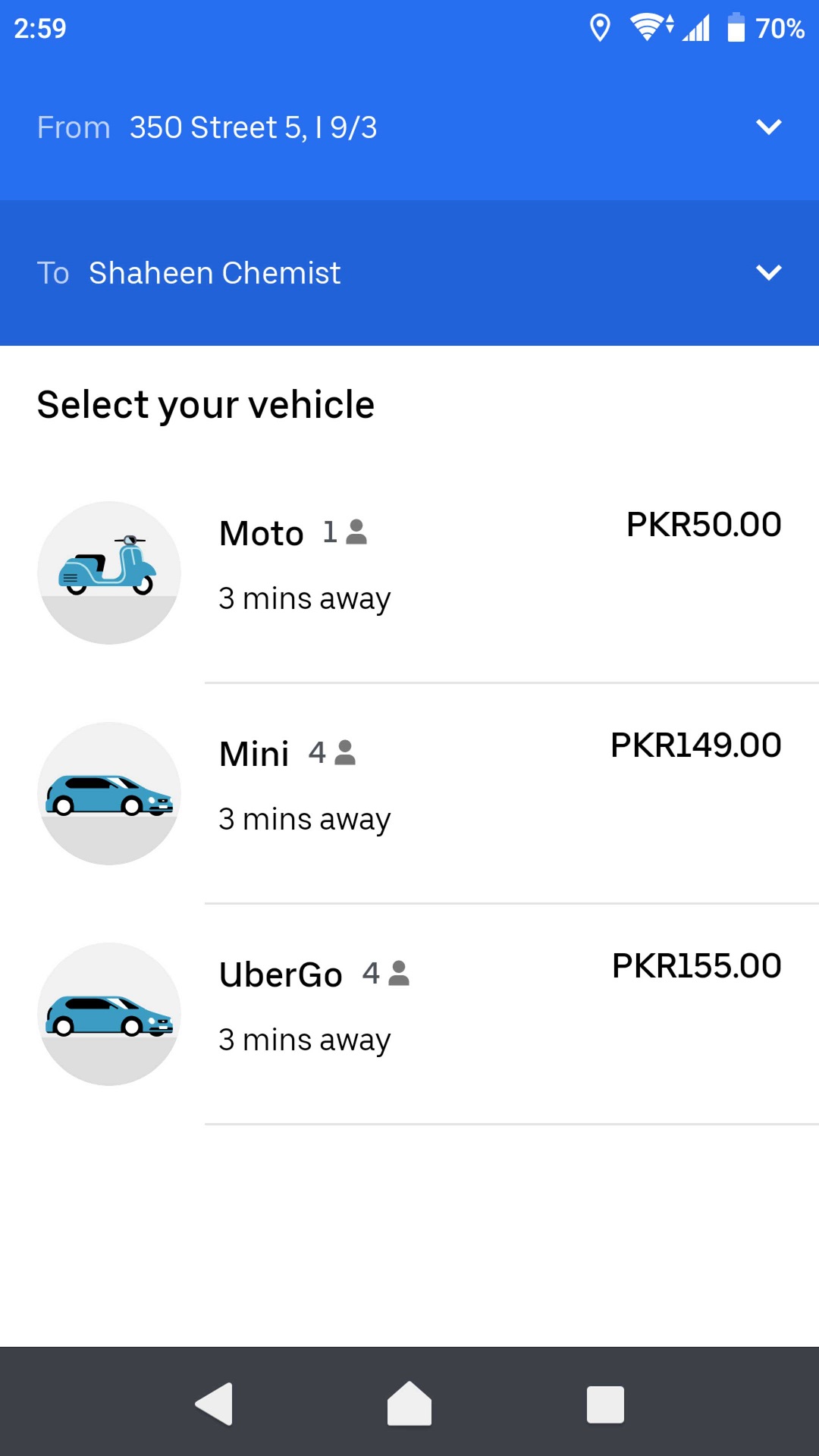This detailed description allows one to visualize the screenshot vividly:

---

A screenshot captures the interface of a ride-sharing app, possibly showing options for renting a vehicle or booking an Uber. At the top of the interface, a blue banner displays the time, "2:59," in white digits. On the left side of this banner, icons indicate the Wi-Fi signal, cellular data strength, and the battery level at 70%.

Below the banner, the screen shows the pickup location, "From 350th Street, 519/3," with a downward arrow beside it. Underneath, it specifies the user's details, "Sue Shaheen, Chemist," also followed by a downward arrow.

The main section of the display features a white background. In bold black text, it prompts the user to "Select your vehicle." The first option shows an icon of a motorcycle or moped labeled "Moto 1." It indicates the vehicle is three minutes away and costs PKR 50.00, suitable for one person.

The next option features an illustrated blue car with dark windows and white tires, labeled "Mini." This option accommodates up to four people, is three minutes away, and costs PKR 149.00. 

A slightly larger car is depicted in the next option, labeled "Uber Go." This car is also for four people, three minutes away, and costs PKR 155.00.

At the bottom of the screen, a black bar contains essential phone navigation icons, including home, back, and recent apps.

---

This caption provides a clear and detailed overview of the screenshot, accurately conveying the visual and textual elements present in the image.